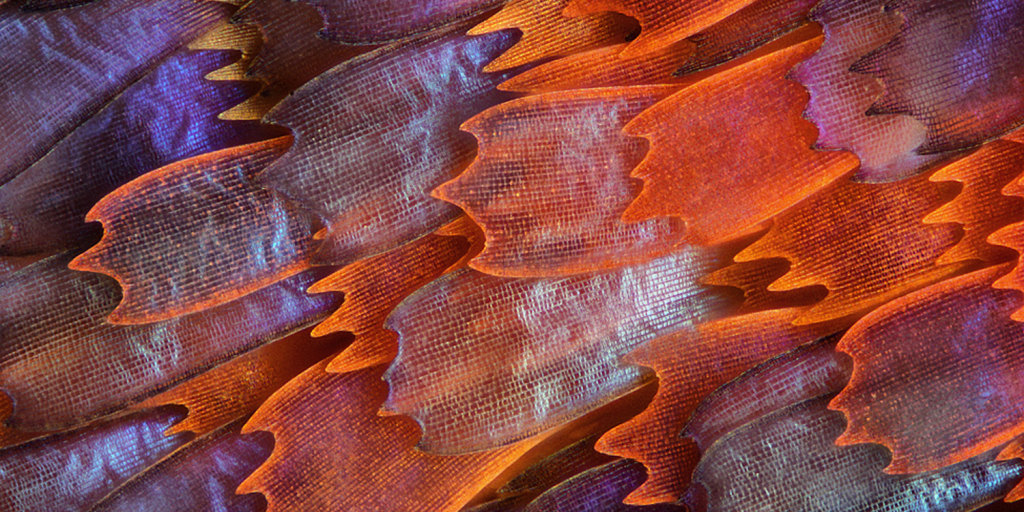The image showcases a highly magnified close-up of the intricately detailed scales of a butterfly wing. The pattern comprises multiple overlapping oval shapes, each adorned with a complex tapestry of fine squares. The color palette spans a variety of hues, including vibrant shades of orange and brown, accented by hints of purple, light blue, pink, and yellow. The scales, reminiscent of the number three due to their three arched curves, create an overall impression of textured, almost reptilian skin. The entirety of the image is dedicated to these repeating shapes, which are magnified 200 times to reveal their mesmerizing details. This captivating shot, an entry by Charles Krebs in the International Digital Imaging Competition, presents a stunning mosaic of the natural world's artistry at a microscopic level, devoid of any background or text.